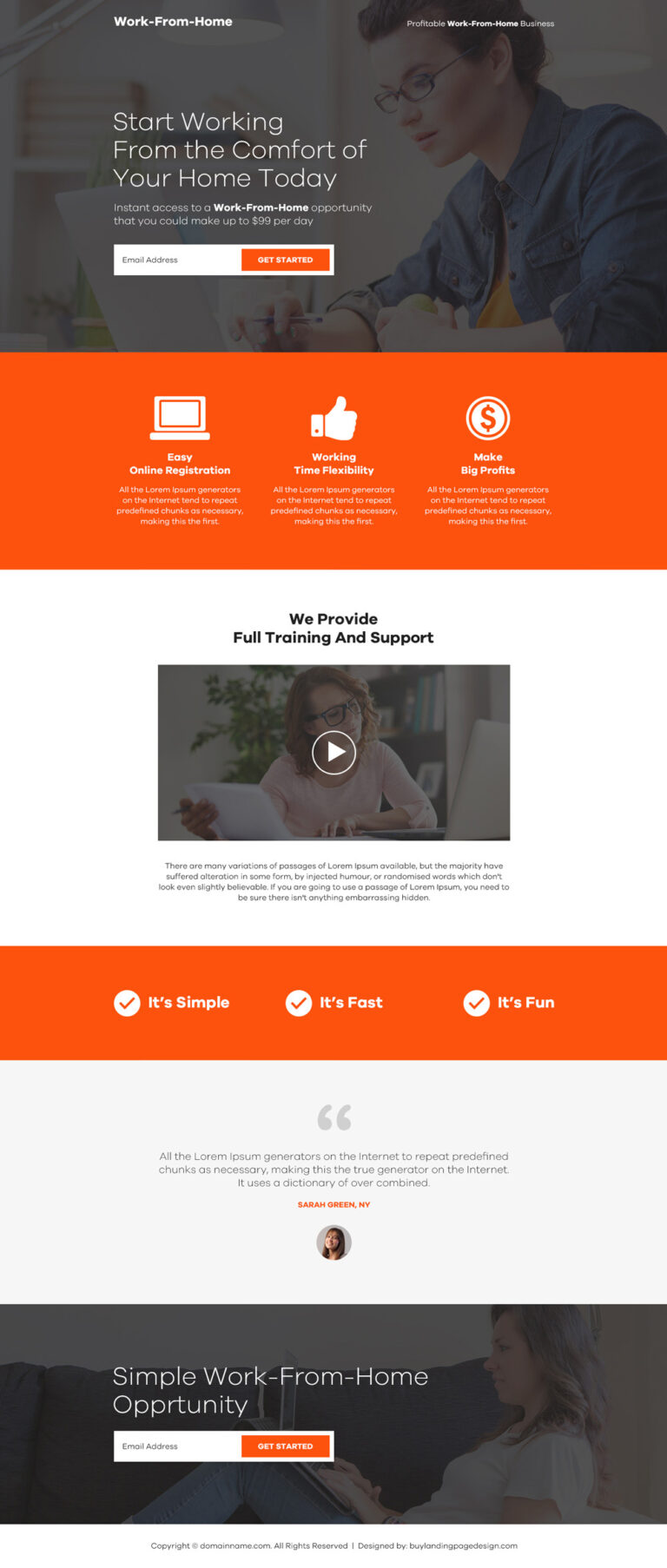The image features a clean, white background with a central picture of a woman sitting at a desk, seemingly in an office setting. The text overlay reads, "Start working from the comfort of your home today." At the top, a search bar with an orange rectangle is prominently displayed. 

Beneath, there's a visual layout including an image of a computer, a thumbs-up icon, and a circle with a dollar sign, each accompanied by informational text. A video thumbnail shows the same woman at her desk, holding an iPad, with a caption that reads, "We provide full training and support."

Further down, an orange rectangle contains three white circles with orange checkmarks, accompanied by the phrases "It's simple," "It's fast," and "It's fun." A quotation and additional information are present, with a person's name in orange text nearby.

On the lower part of the image, a profile circle features the same woman's picture, and another image shows her sitting on the floor with an iPad. The text "Simple Work-from-Home Opportunity" stands out on the side. The image also includes both white and orange rectangles with white text that is hard to decipher, along with a final line of information at the bottom.